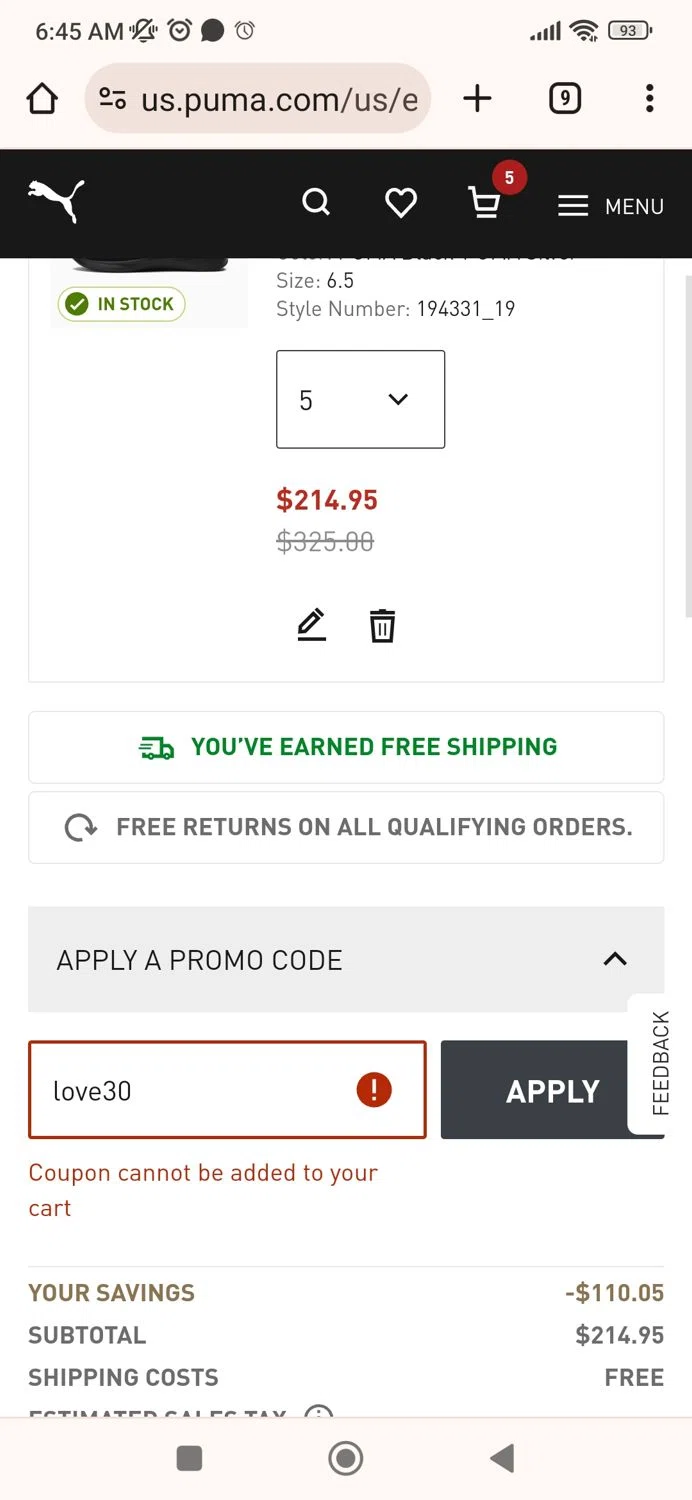Screenshot of a Puma.com Checkout Page:

The screenshot captures the checkout page of the Puma.com website, accessed through a mobile phone at 6:45 AM. The phone has full signal strength, Wi-Fi connectivity, and shows a 93% battery level. An alarm is set but is currently off, and there is a recent text message notification present. The browser has nine tabs open, with the current tab being the Puma shopping cart page.

At the top of the webpage is the Puma logo, displayed as a white graphic on a black background. Next to the logo are icons for search, likes, and the cart, which contains five items. The contact menu is listed as "Menu."

The shopping cart details show that five identical items, listed as style number 194331_19 in a size 6.5 and in red, have been added to the cart. The initial total was $325.00, but a reduction to $214.95 suggests a promo code or discount has already been applied. There is a message confirming that the customer has earned free shipping, indicated with a green truck icon and the text "Free Shipping."

Additionally, there is the option to apply another promo code. The user attempted to enter the code "LOVE30" by tapping the black 'Apply' button, but a message indicates that "Coupon cannot be entered to your cart." The savings amount is displayed as $110, bringing the subtotal to $214.95. The shipping cost is listed as free, while the estimated sales tax amount is cut off and not entirely visible.

At the bottom of the screen, there are the standard home menu, contacts menu, and back button options. A feedback button overlaps with the promo code application section, adding some clutter to the interface.